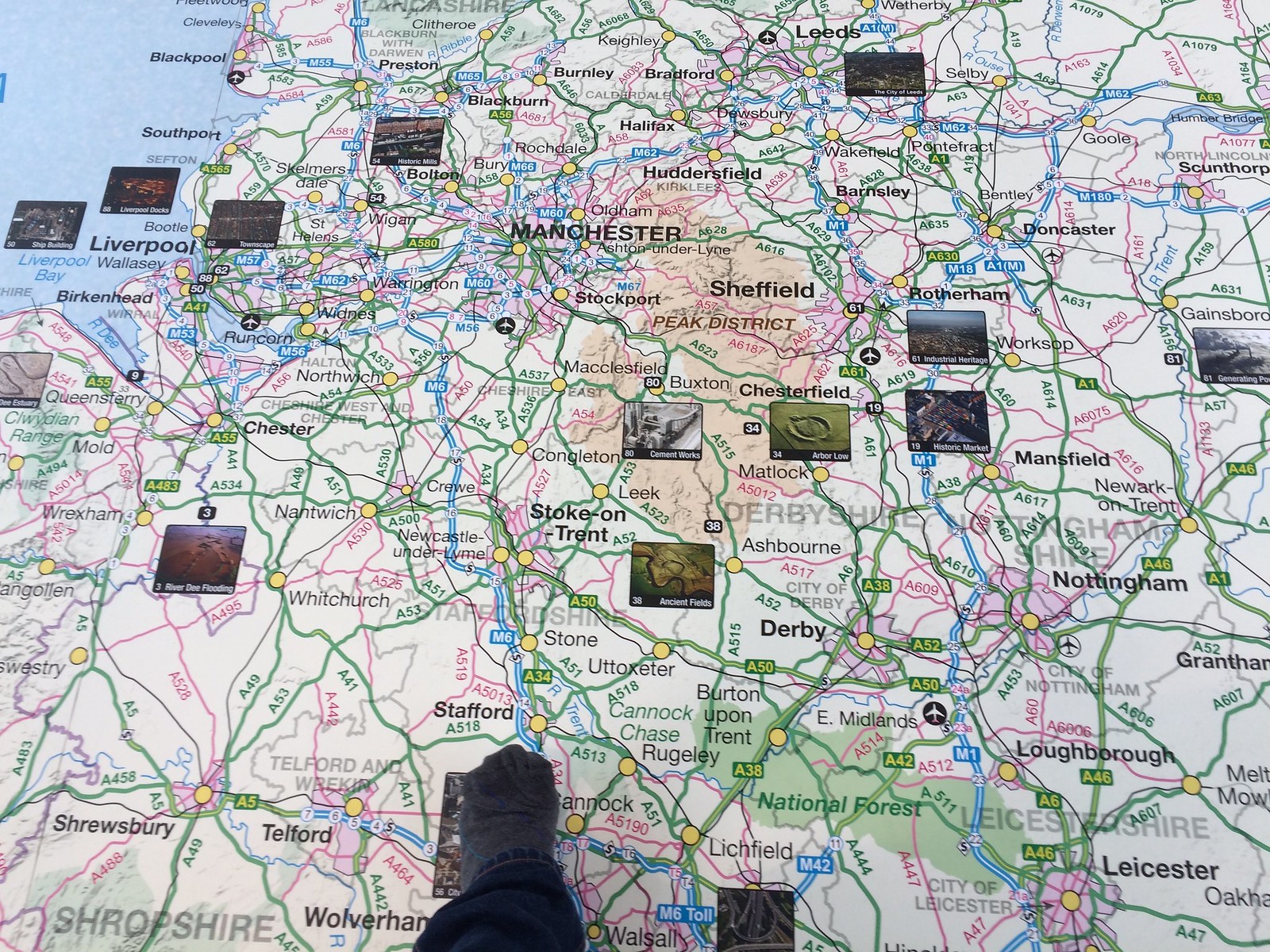This vibrant color photograph features a detailed map of a portion of Northern England, with Manchester prominently positioned near the center. The map highlights major cities including Liverpool to the west, Sheffield and Derby to the south, Stafford and Telford further west below Stoke-on-Trent, and Leeds at the very top center. On the map, various colorful squares, each containing tiny images and numbers, are strategically placed over different areas. Notably, one square near Stoke-on-Trent bears the number 38 and a label, "ancient fields".

To the right, cities such as Leicester, Nottingham, and Mansfield are marked, while Doncaster is found further north near Leeds. Smaller towns like Rotherham, Shrewsbury, Wolverham, Chester, Birkenhead, Lowborough, and Whitechester are also indicated. The image conveys a sense of active engagement with the map, as a person's hand is visible at the bottom, seemingly affixing the numbered squares, and a foot steps onto the map, suggesting it might be laid out on the floor.

Bright colors, including blues, greens, pinks, and yellows, demarcate various regions and roads across the map. The intricate details, with notable locations and pictorial representations, capture the essence of this northern region of England, making it a focal guide to key cities and landmarks.